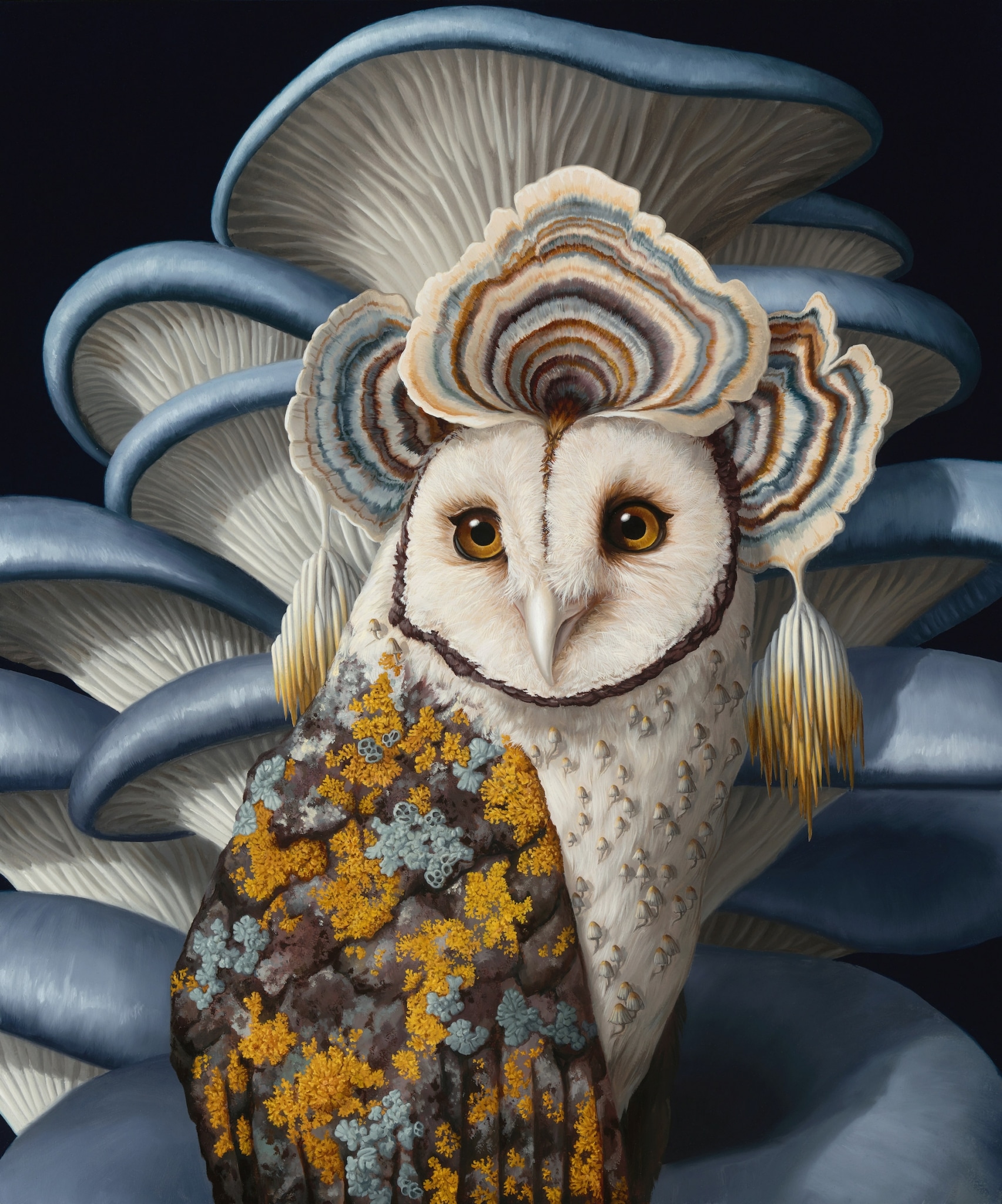The image depicts a hyper-realistic painting of a snow owl against a black background, showcasing incredible detail and artistry. The owl’s white face contrasts sharply with its striking hazel brown eyes and a sharp white beak. Extending from under its chin is a colorful shroud that resembles floral decorations in shades of blue, gray, and yellow, draping down like an elegant robe.

The owl's chest is predominantly white but features intricate, raised portions that create a sense of textured depth. Surrounding and behind the owl is an array of mushroom spores, depicted in soft, squishy forms with blue, light blue, and gray hues. These fungal elements form a backdrop that adds an ethereal quality to the piece, almost appearing as a mountain of mushroom spores encircling the owl.

Additionally, the owl has shell-like shapes positioned above its head and around where its ears would be, enhancing the mystique of the portrait. Multicolored circular objects hover above, blending gold, brown, and light blue hues, and a large blue border frames the lower part of the image, setting the owl into the scene with a dreamlike placement. The absence of any text allows the viewer's focus to remain solely on the stunning, lifelike details that highlight the painting's professional craftsmanship.